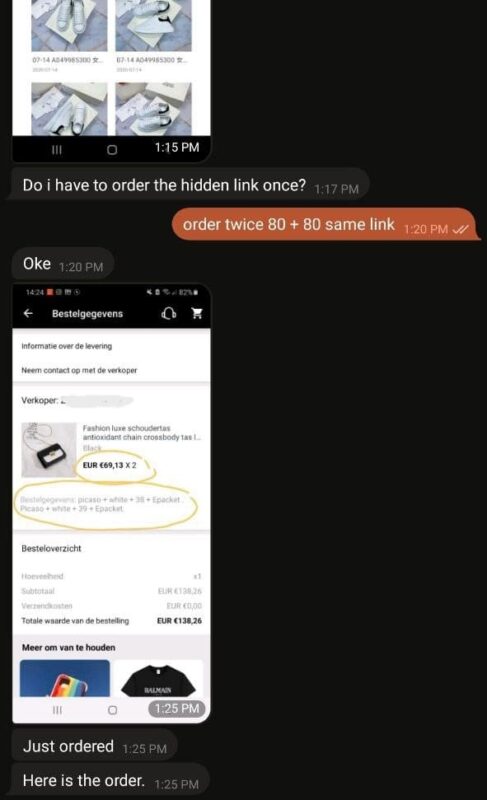The image depicts a conversation between individuals within a texting app, formatted to look like a smartphone or tablet screenshot. At the top of the image, there are four photographs showcasing a pair of grey sneakers that have a silver-like appearance. Below the images, there's a bezel displaying four lines and a circle, along with a timestamp indicating "1:15 PM."

The first message in the conversation reads, "Do I have to order the hidden link once?" with a timestamp of "1:17 PM." The response, marked in orange text, reads, "Order twice, 80 plus 80, same link," followed by two check marks indicating the message has been read, with a timestamp of "1:20 PM." Following this, the reply "OKE" appears in white text, also timestamped "1:20 PM."

The subsequent segment shows another screenshot, featuring a URL accompanied by a white arrow, the word "bestelgegevens," a headset icon likely for chat support, and a shopping cart icon. The text continues in a different language, stating "Information over de-leveling" and listing details such as "Name, Contact, OP, met, de recouper." Additionally, it shows "euro, 69,13 times X," which is circled, along with another section indicated within the screenshot. Finally, the conversation concludes with the message, "Just ordered at 1:25 PM. Here is the order," timestamped "1:25 PM."